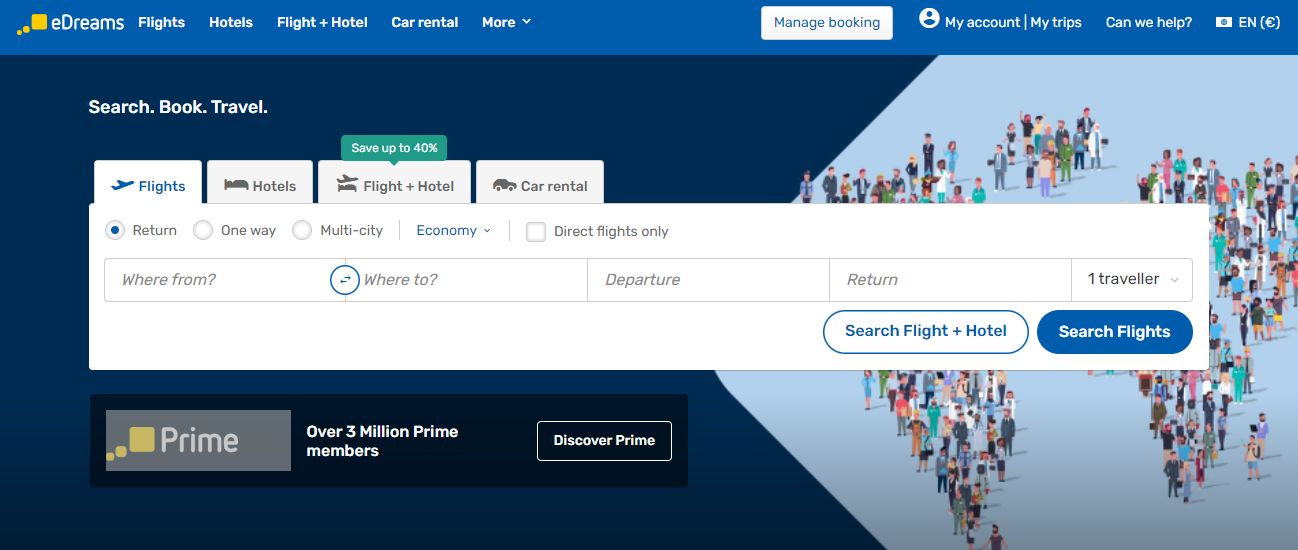This is an image showcasing the homepage of the eDreams website. In the top left corner, there is a distinctive yellow icon composed of two small yellow circles followed by a yellow square. To the right of this icon, the brand name "eDreams" is prominently displayed.

Across the header, there are several navigation tabs. From left to right, they read: "Flights," "Hotels," "Flight + Hotel," "Car Rental," and a "More" option indicated by a downward-facing arrow.

On the top right, additional tabs are available, providing users with options such as "Manage Bookings," "My Account," and "My Trips." Further to the right, there is a "Can We Help?" section followed by the language selection "EN."

Below the header, a tagline reads "Search. Book. Travel." Providing guidance to users. There are more navigation options just below this tagline, with tabs labeled from left to right as "Flights," "Hotels," "Flight + Hotel," and "Car Rental." Above these tabs, a promotional banner advertises savings of up to 40%.